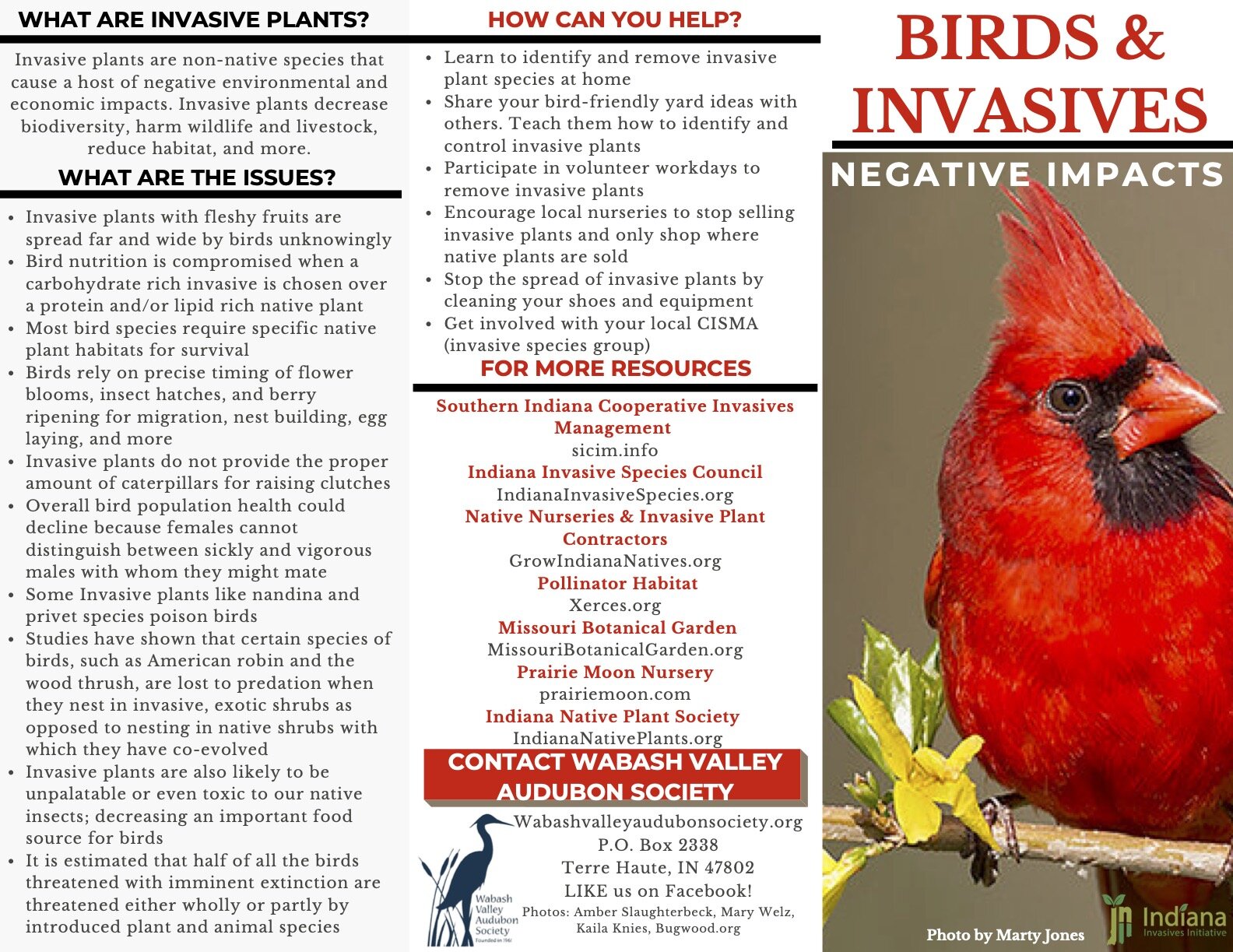The image is an informative insert from an article about birds and invasive species, set against an all-white background. It contains four sections, each with a specific focus. The top-left section is titled "What are Invasive Plants" in black lettering and has a detailed insert explaining the concept. Below it, another section titled "What are the Issues" also in black lettering, discusses the various negative impacts of invasive species on birds and native plants.

The central section, highlighted with red lettering, is titled "How Can You Help" and lists different actionable ways individuals can contribute to mitigating the impact of invasive species. Immediately below is another section in red lettering titled "For More Resources," which provides contact information for organizations that offer assistance.

A prominent red banner with white text at the bottom announces, "Contact Wabash Valley Audubon Society," accompanied by mailing information and an image of a pelican standing next to some grass. On the right side of the insert, there is a colored photograph of a cardinal perched on a tree branch with a flower, credited to Marty Jones in Indiana. The cardinal photo draws attention to the real-life impact of invasive species on local bird populations.